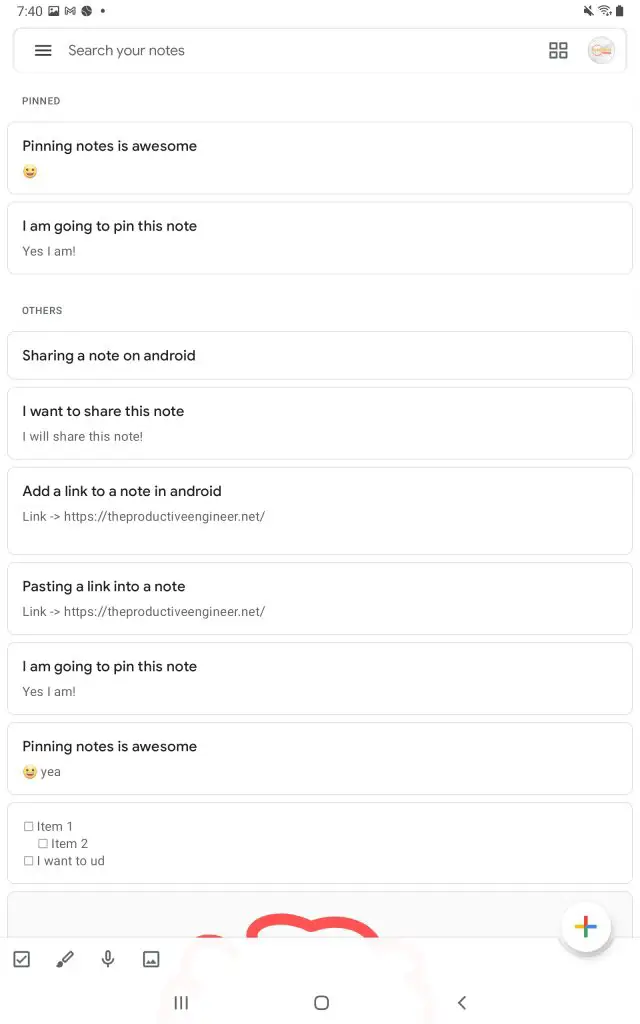In this image, we see a screenshot of a mobile phone displaying the interface of a note-taking application. 

At the very top, the status bar shows the current time on the left, a strong Wi-Fi signal indicator, and the battery icon to the right. Below this, there is a rectangular search bar featuring a menu icon, the text "Search your notes," and the Microsoft logo, which might also denote a categorization feature.

The main content begins with a section labeled "Pinned," which includes a rectangular box. Within this box, the text "Pinning notes is awesome" is prominently displayed, accompanied by a smiling emoji directly below the text.

Following the "Pinned" section, we encounter another rectangular white box containing the text "I'm going to pin this note" in black font, then "yes, I am!" in gray font with an exclamation mark emphasizing the statement.

Next, there is a category marked "Others," under which several notes are listed. The first note box reads "Sharing a note on Android" in black text. The subsequent note states, "I want to share this note. I will share this note!" also in black text, emphasizing the declaration with an exclamation mark. Another note in this category is titled "Add a link to a note in Android" with the associated hyperlink beginning with "HTTPS."

Additionally, there is a note indicating the action "Pasting a link into a note," and yet another box reiterating the text "I am going to pin this note," similar to the one found earlier in the "Pinned" section. Finally, a repeated note highlights "Pinning notes is awesome," along with a smiling emoji once more.